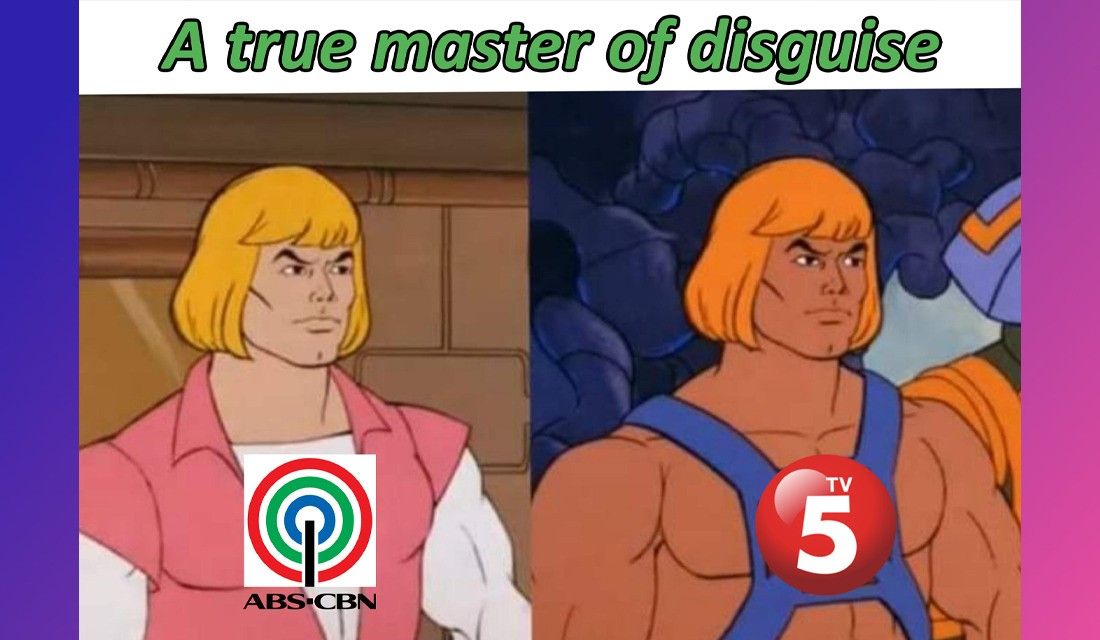The image is a cartoon depiction of two different forms of the character He-Man, placed side by side under the greenish text "A True Master of Disguise." On the left, He-Man dons his iconic blonde bob cut, a pink vest with a white skin-tight undershirt, and his menacing gaze directed to the right. Over his chest is an ABS-CBN logo, characterized by three concentric circles in red, green, and blue, surrounding a vertical black line. This image shows He-Man standing inside a building with a brick wall and a window behind him, framed by a dark blue vertical border on the far left.

On the right, the second image features He-Man with slightly darker blonde hair and a tanner skin tone, showing off his muscular, shirtless physique with blue straps across his chest. This version has a TV5 logo prominently displayed on his chest, marked by a red circle with the TV5 label inside it. The background behind this He-Man is a non-descript gray blur, accompanied by the partially visible armor of another character, Men-At-Arms. The right side of the composition is bordered with a pink-purple vertical band.